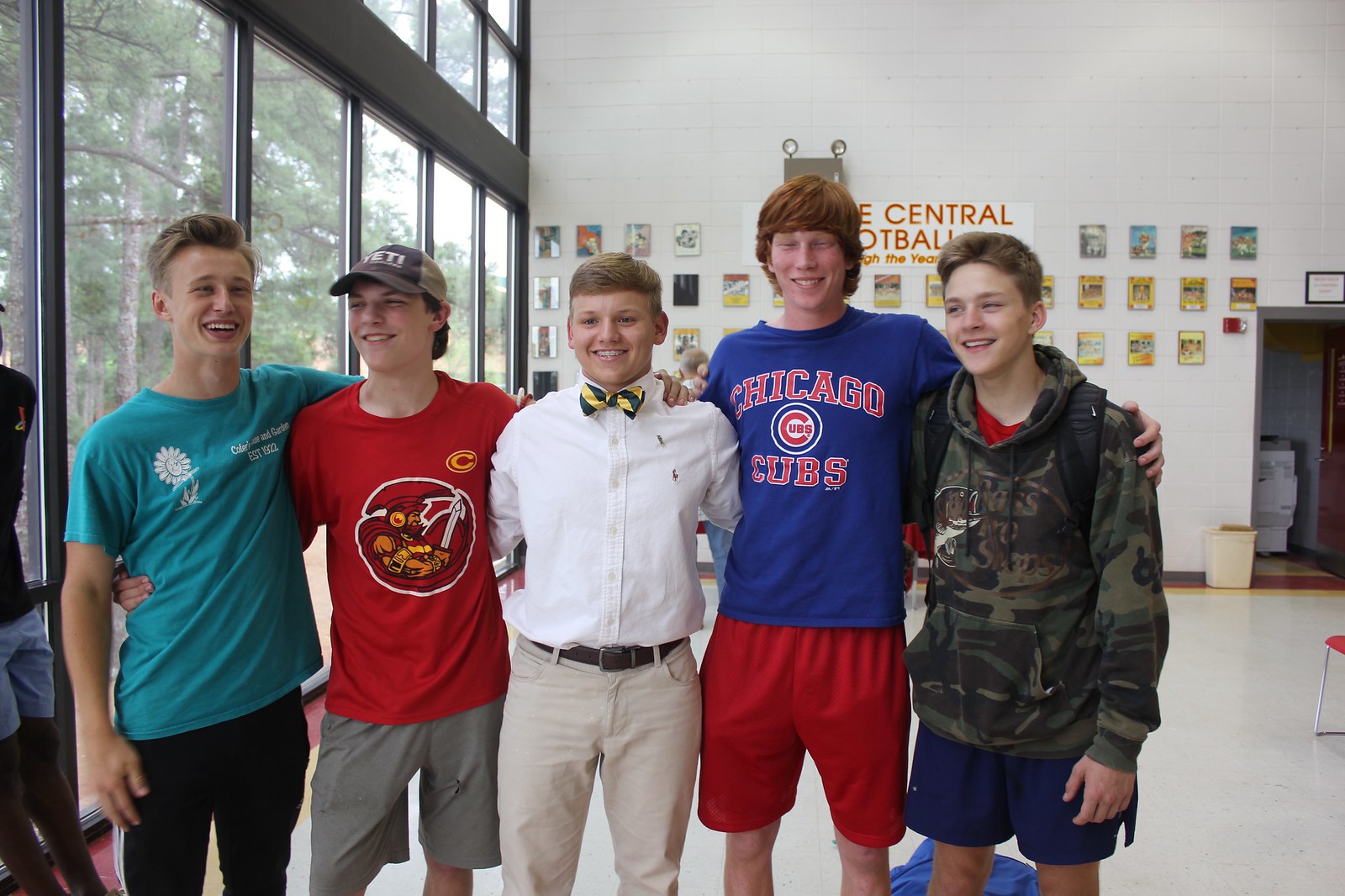This image captures a group of five high school boys standing shoulder to shoulder with their arms around each other, suggesting a strong camaraderie among them. They are positioned slightly to the left, facing the camera directly. The boy on the far left is wearing a blue t-shirt with black pants, next to him is a boy dressed in a red t-shirt with gray shorts. In the middle stands a shorter, slightly nerdy-looking boy in a white button-down shirt paired with beige khakis and a green and gold striped bow tie; his short blonde hair and toothy smile give him an endearing look. To his right is a red-haired boy in a bright royal blue Chicago Cubs t-shirt with red shorts. The last boy on the far right is wearing a green camouflage sweatshirt with blue shorts, potentially a Yeti hat as well. The boys are set against a background showing a high-ceilinged school building with white walls adorned with hand-sized photos, likely of football players and leading figures. Behind them, you can also see silver-framed windows revealing green and brown trees. An open door with a trash can beside it is visible on the far right, next to the artwork that decorates part of the wall. The overall scene exudes a youthful, school spirit with casual yet diverse attire among the group.